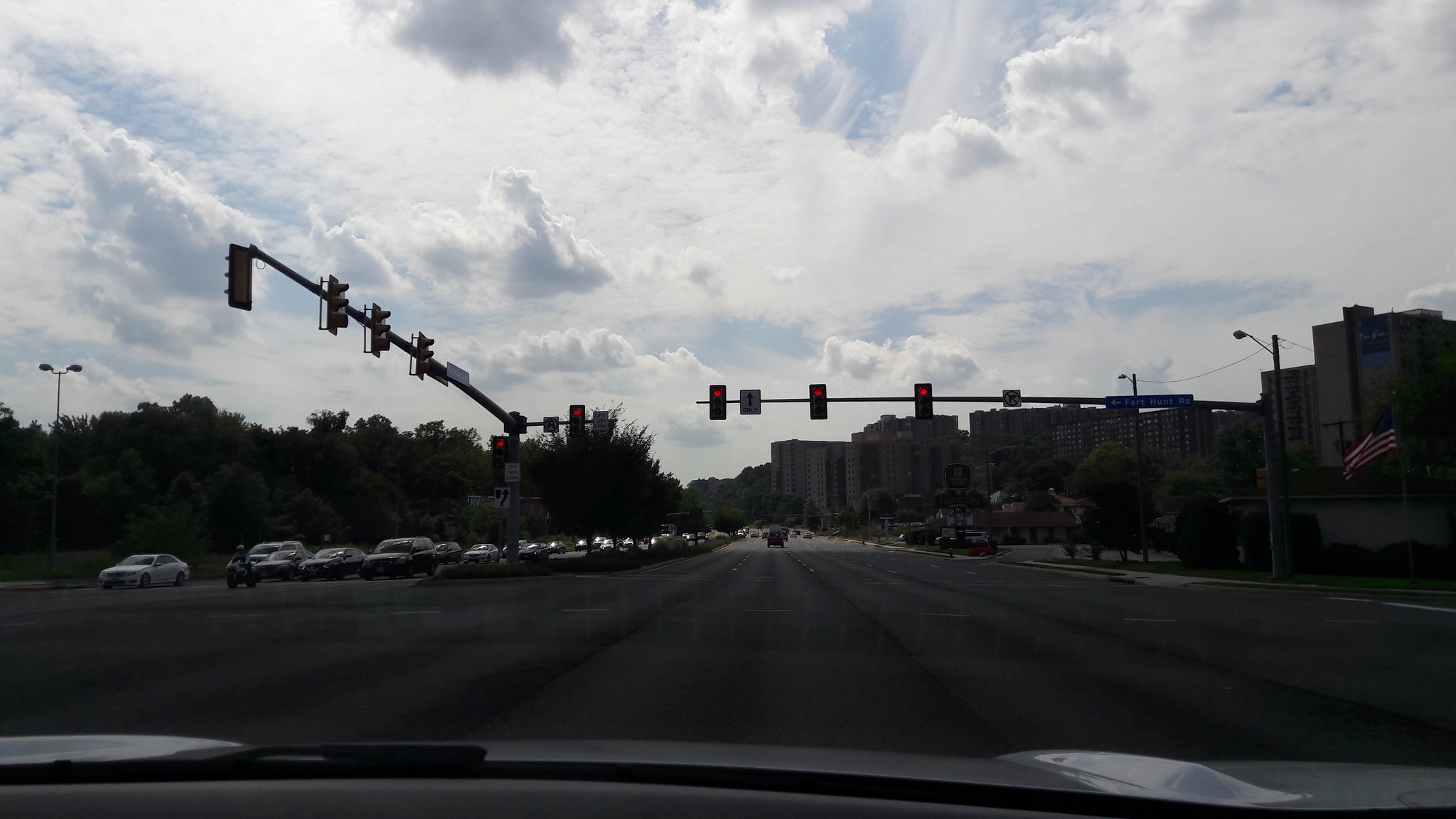This photograph captures a street scene at dusk, taken from inside a car halted at a red light. The scene reveals cars that have already passed through the intersection ahead, with additional vehicles stopped at the light headed in the opposite direction. The sky, exhibiting lingering hues of blue and white clouds, contrasts with the early evening darkness that envelops the surroundings. The predominant colors are the red of the traffic lights and the subtle tones of the sky, while the rest of the scene is muted in gray and dark shades, enhancing the tranquil yet urban ambiance of the moment.